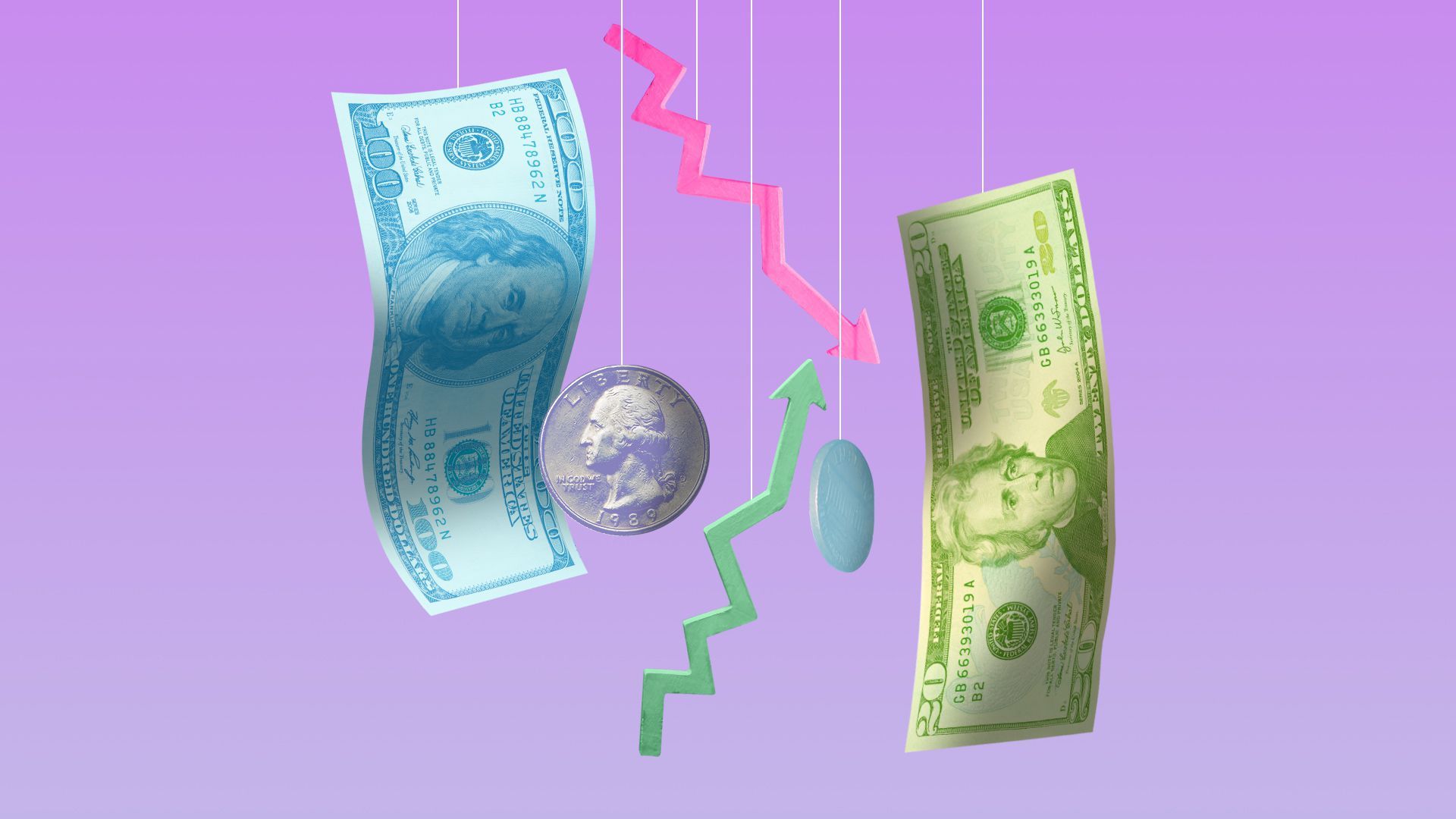This rectangular landscape image, adorned with a lavender background, resembles a clip-art style mobile and represents the dynamics of the stock market and investments. The image, which is much wider than it is high, features six thin white strings of varying lengths descending from the top. 

On the far left, a slightly curved $100 U.S. bill featuring Benjamin Franklin, distinguished by its light bluish hue, hangs from one string. Adjacent to it and descending from a longer string, a 1989 U.S. quarter showcases the head side with George Washington. In the center, two jagged arrows dangle: a shorter string supports a red arrow pointing downward, while the longest string in the display holds a green arrow pointing upward.

On the right side, a $20 U.S. bill featuring Andrew Jackson is oriented at a 90-degree angle. Between this bill and the center arrows is a mysterious blue coin-like object, which does not appear to be actual currency. The overall layout, with its combination of currency and directional arrows, evokes the fluctuating behaviors of stock market trends.